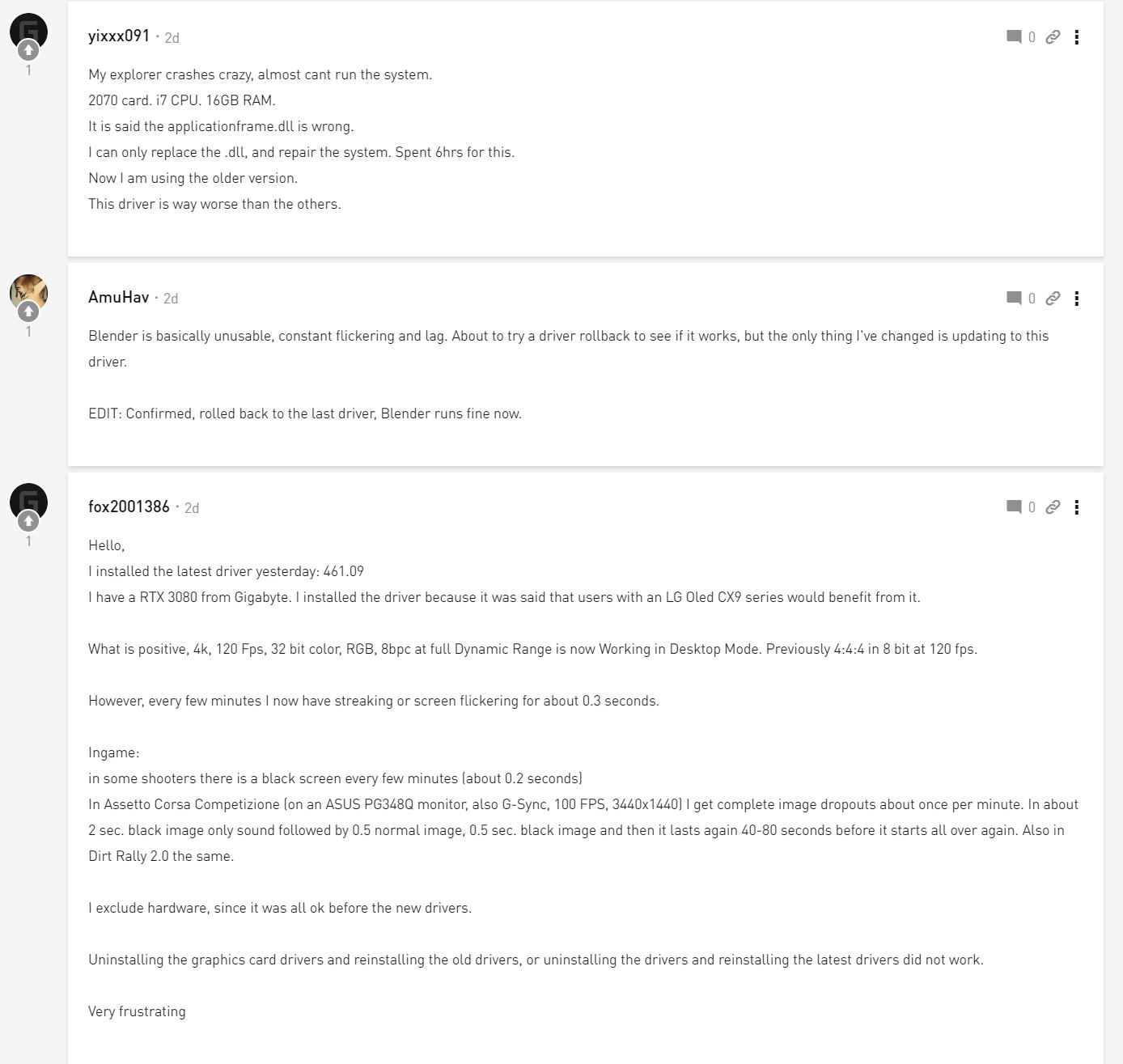The image depicts a computer screen displaying an online conversation among several users discussing technical issues with their graphics drivers. On the left side, there are icons, possibly representing different applications or users, while the main conversation text is centered in the middle of the screen.

- User yix091 comments: "My Explorer crashes constantly; I can hardly run the system. It mentions a 2070 card and something with RAM. There's an error with the application frame.dll. I had to replace the dll and repair the system, which took six hours. Currently, I'm using an older version of the driver, which is much worse than the previous ones."

- User amuhav responds: "Blender is extremely unstable right now, with constant flickering and lag. I'm planning to try rolling back the driver to see if that fixes the issue. The only change I've made recently is updating to this new driver." Later, they add: "Confirmed, rolling back to the previous driver fixed the issue. Blender runs fine now."

- Another user, Fox (followed by several numbers), chimes in with a lengthy response about installing the latest driver and expressing their frustration with the ongoing technical problems.

Overall, the conversation illustrates the users' shared frustration with the instability caused by the new graphics driver and details their troubleshooting efforts, including driver rollbacks, system repairs, and hardware issues related to RAM and a 2070 graphics card.